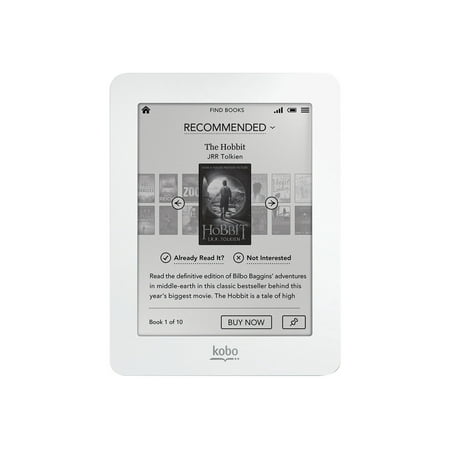The image showcases a white Kobo e-reader with a completely white background. The Kobo logo, in lowercase letters with an underscore beneath it, is prominently displayed on the bezel at the bottom of the device. The screen features a menu bar at the top, displaying a home icon on the left, and indicating "FIND BOOKS" in all caps in the center. To the right are Wi-Fi signal bars, a battery icon, and another unidentified icon, possibly in a hamburger menu style.

The main portion of the screen highlights a recommendation for "The Hobbit" by J.R.R. Tolkien. The word "RECOMMENDED" is in all caps at the top, followed by the title and author's name beneath it. An image of the book cover occupies the central area of the screen. Below the cover, there are interactive options: on the left, buttons for "ALREADY READ IT" or "NOT INTERESTED," and on the right, buttons to navigate left or right, presumably to browse more books.

Further down, a descriptive text starts with "READ THE DEFINITIVE EDITION OF BILBO BAGGINS' ADVENTURES IN MIDDLE-EARTH. In this classic bestseller behind this year's biggest movie, THE HOBBIT IS A TALE OF HIGH-" but the rest is cut off. Near the bottom-left of the screen, it says "BOOK ONE OF TEN." A "BUY NOW" button in all caps is located to the right, next to a pushpin icon button.